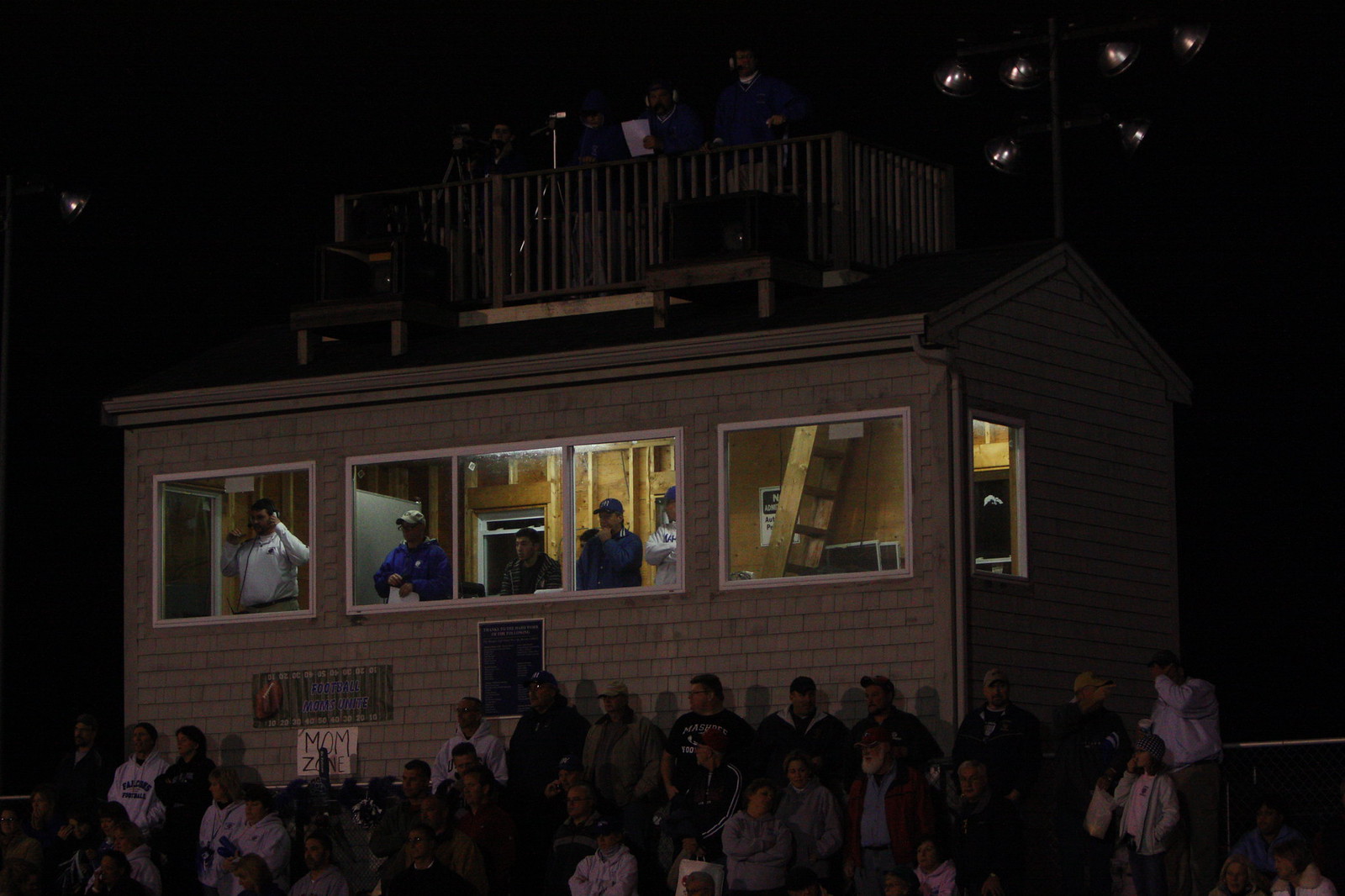This is a colored photograph taken outdoors at night, likely at a football game during a chilly fall evening. The scene is illuminated by outdoor stadium lights visible at the top right corner. In the foreground is a small, light brown brick, ranch-style building with a deck built on its roof. The deck is occupied by several men; one appears to be holding a camera, another is carrying a piece of paper, and a couple are wearing headphones, suggesting they are involved in coaching, officiating, or announcing the game. Below the deck, inside the building, more men are visible, most of whom are wearing headphones and appear to be intently focused, likely engaged in taking stats or calling the game. Surrounding the building, the stands are filled with fans, most of whom are bundled up in sweatshirts or jackets. The overall scene captures the dynamic atmosphere of a nighttime sporting event, highlighting both the activity within the broadcast or coaching booth and the engaged spectators.